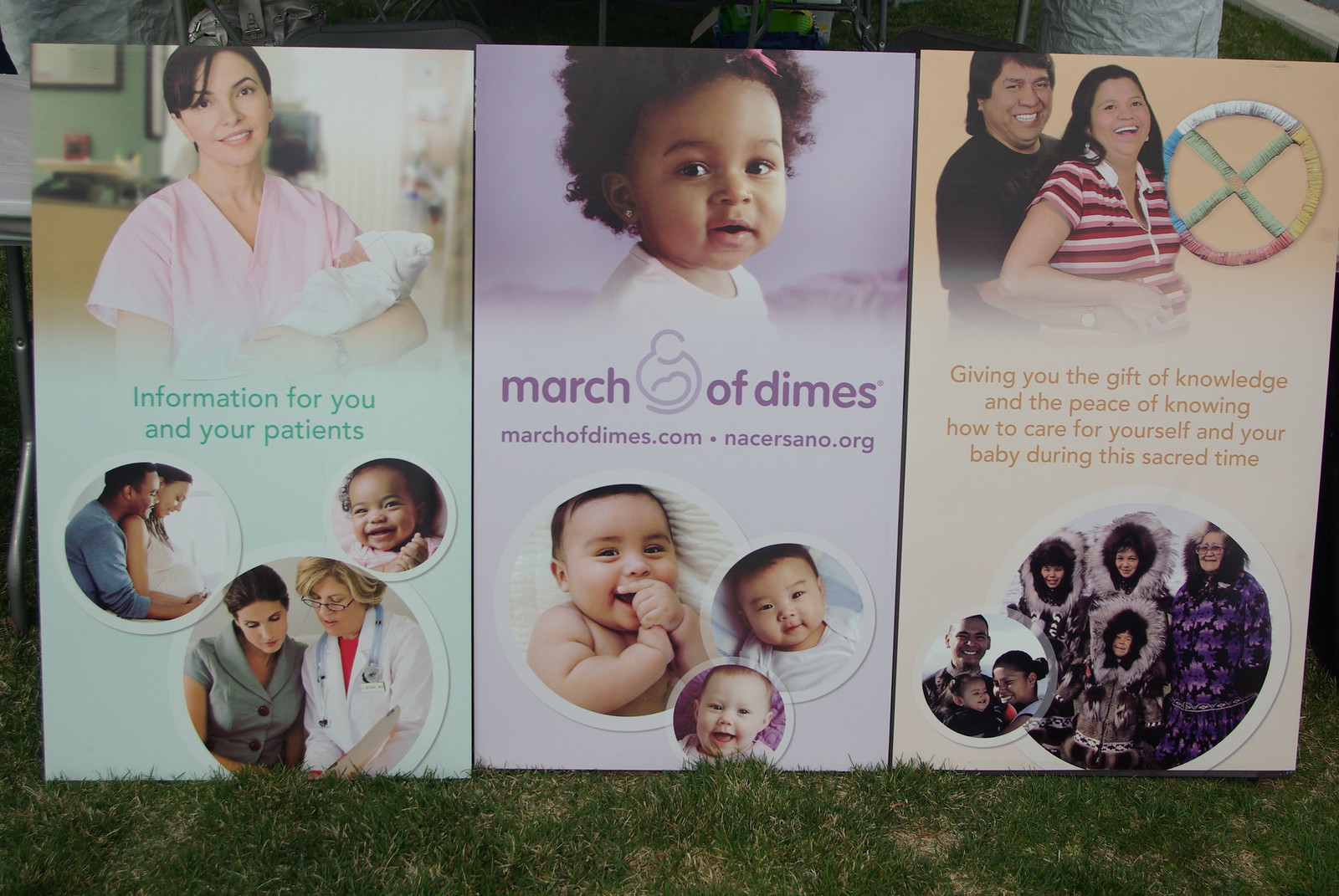The advertisement consists of three upright panels placed on a grass ground. The left panel, set against a light green background, features the heading "Information for you and your patients." At the top, it shows a woman cradling a baby, and below this are three circular photographs: one of a couple, one of a woman consulting with a doctor, and one of a baby. The central panel, with a purple background, displays the text "March of Dimes" and the URLs "marchofdimes.com" and "nacersano.org" in violet color below a photograph of a small baby or young child. Beneath this are three more circular pictures, each depicting a different baby. The right panel, also set against a light green backdrop, reads "Giving you the gift of knowledge and the peace of knowing how to care for yourself and your baby during this sacred time." At the top, it features a photograph of a laughing couple, next to a circle with a cross inside. Below this are two circular images: a smaller one showing a couple with a child, and a larger one depicting four people, some of whom appear to be wearing heavy coats.